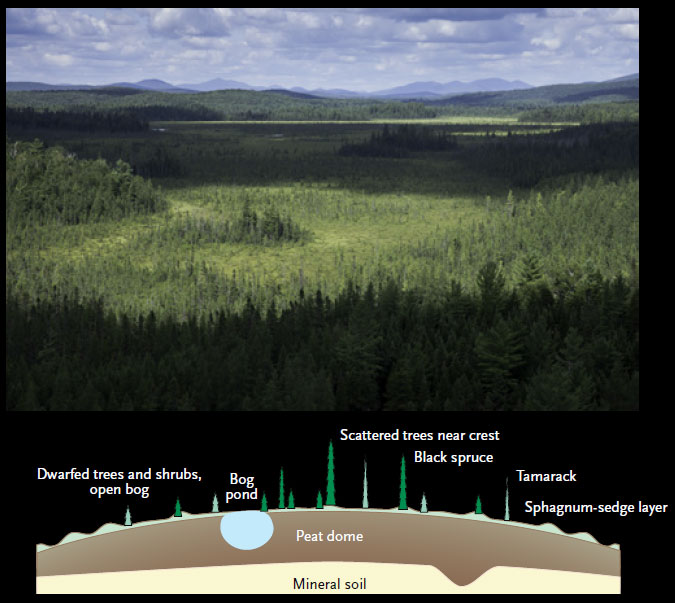The image comprises two sections: the top features a photograph of a sprawling forest with dense trees flanking a slight valley that has fewer trees. The background reveals foothills under a cloudy sky. Below the photograph, an animated cross-sectional diagram details the soil strata and vegetation of the depicted landscape. The diagram illustrates the Earth's curvature and starts with mineral soil at the bottom, overlaid by a peat dome. At the very top layer, labeled the sphagnum sedge layer, various vegetation types are identified. On the far left, the diagram highlights dwarf trees and shrubs in an open bog area, next to a blue circle representing a bog pond. Further to the right, the illustration shows scattered trees near the crest, including black spruce and tamarack.